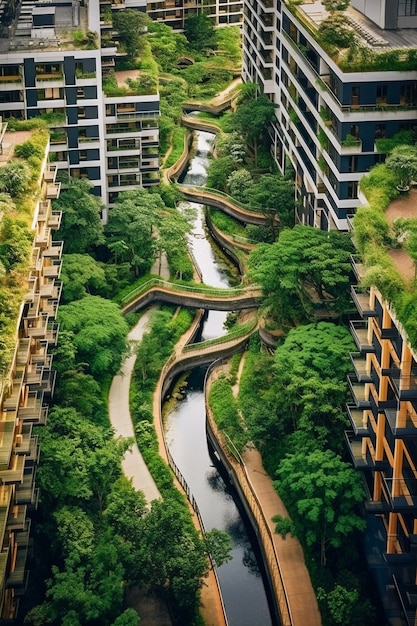The image depicts a futuristic or possibly abandoned cityscape captured in portrait mode, towering over urban structures that are approximately seven to eight stories high. From a vantage point at least twice the height of the buildings, the scene reveals a winding, man-made river running through the center, flanked by a walking path on each side colored in hues of light brown. Numerous bridges interconnect over the river, which is serene and free of any floating debris, indicating a stillness that complements the absence of human activity.

The city appears suffused with nature's reclaim, as lush greenery, trees, and bushes proliferate not only along the riverbanks but also on the rooftops of apartment-like buildings. These buildings, resembling condos or hotels, are characterized by their symmetrical architecture and commonly feature off-white to light brown exteriors with balconies. Despite the aesthetic coherence and sunny, well-lit ambiance, the area feels deserted, with no sign of human presence. The overgrown vegetation and unkempt walkways emphasize a sense of abandonment, suggesting that nature has gradually taken over the once-maintained urban landscape.